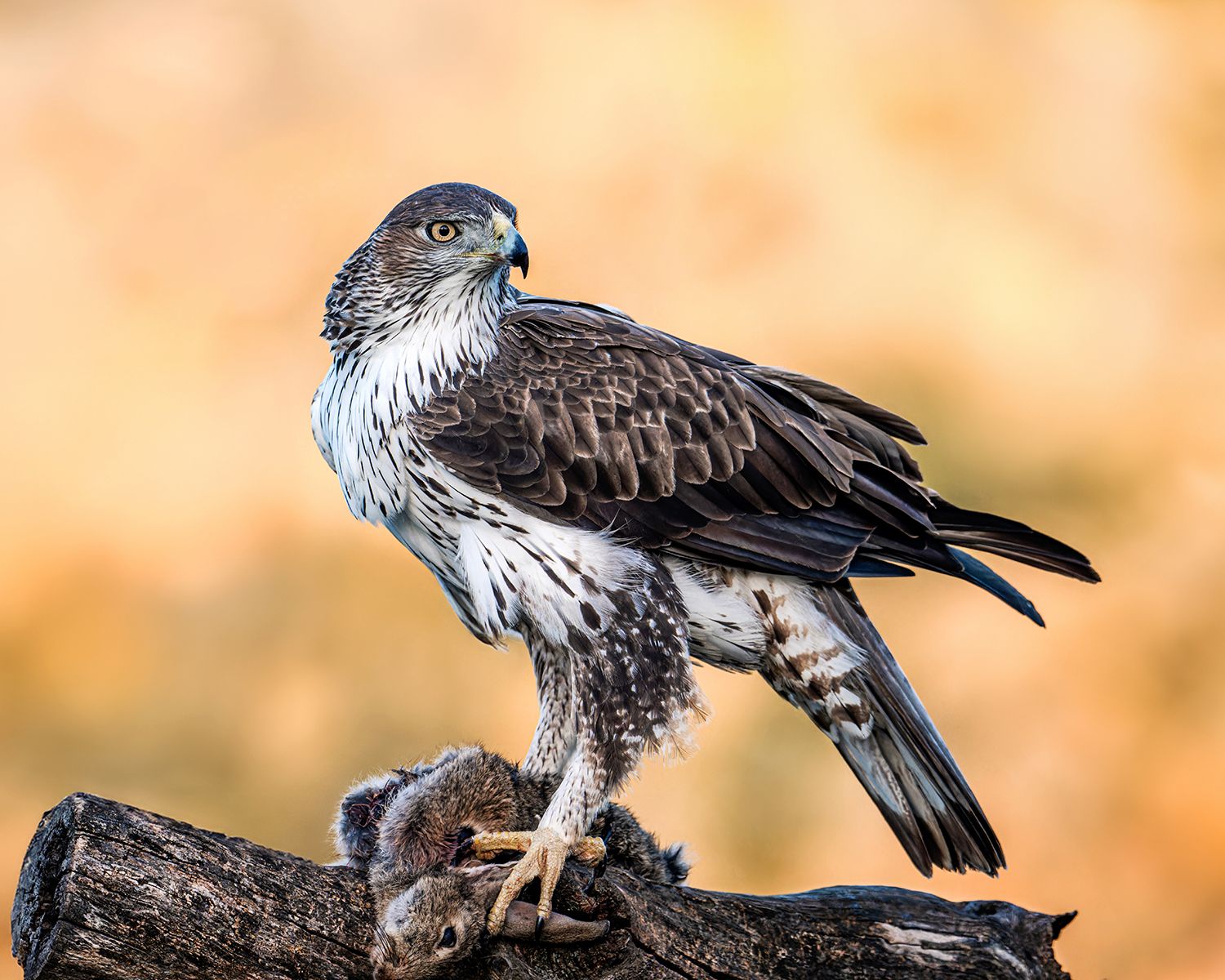The image depicts a professional photograph of a dark gray hawk with an array of feathers, perched on a log in its natural habitat. The hawk's strong yellow talons grasp a dead rabbit, likely captured as prey. The background is an out-of-focus brown-orange, creating a stark contrast that emphasizes the bird's sharp features. The hawk's body is oriented to the left while its head twists to the right, showcasing piercing light yellow eyes and a black, downward-hooking beak. The belly of the bird is white with black speckles, adding to its intricate feather pattern. This striking image, reminiscent of a National Geographic capture, highlights the fierce grace of the hawk as it surveys its surroundings.